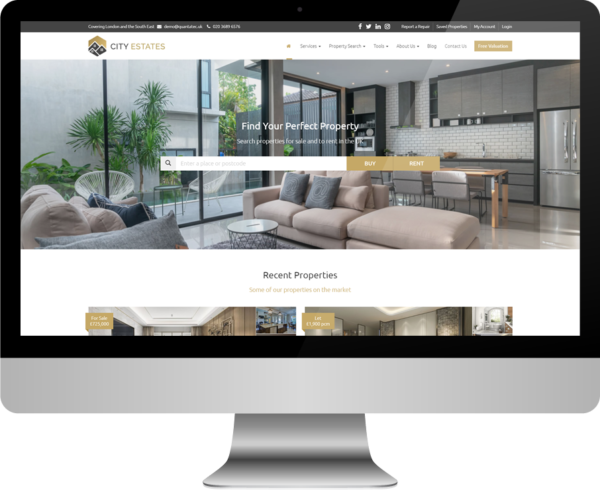The image portrays a sleek, silver computer monitor with a reflective finish. The design features a long, thin, curved silver stand and a silver base, with black bezels framing the display. On the screen, the monitor displays a website titled "City Estates," prominently located in the top left portion on a white banner. The website's logo resembles a diamond shape with black mountains in the background. 

Navigation links with dropdown menus are also visible across the top banner. The centerpiece of the site is a striking photograph of a modern, elegant house with abundant glass, bright interiors, light-colored furniture, stone floors, and silver kitchen appliances. The generous windows reveal lush green trees outside. Additionally, there's a search box allowing users to filter property listings by choosing "Buy" or "Rent" options.